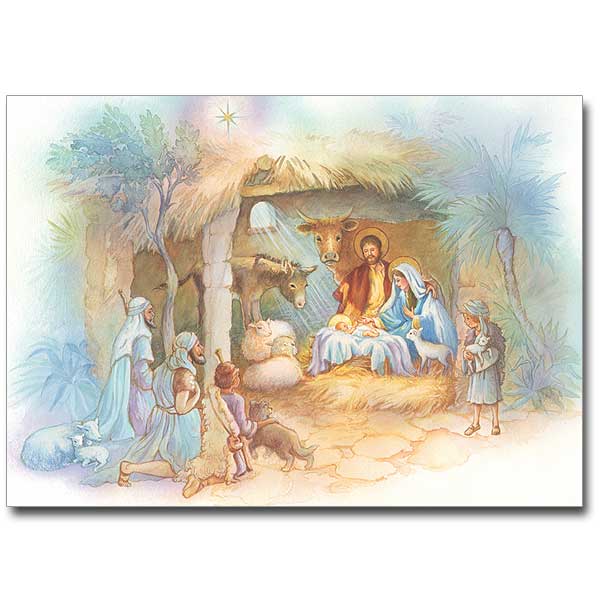This hand-drawn, colored pencil depiction of the nativity scene captures the serene and divine moment of Jesus' birth with intricate details and soft, natural colors like light green, blue, and purple. At the heart of the scene, baby Jesus lies in a manger within a humble stable. Mary sits closely over him while Joseph stands by her side, with his hand gently placed around her. The gentle glow of the North Star above shines through the hut's window, illuminating the newborn.

Surrounding the Holy Family, the animals add a rustic charm: a cow and a donkey gaze lovingly at baby Jesus, while two sheep, one lying down, observe quietly. On the bottom left, the three wise men kneel with gifts, one holding a dog beside a lamb with its baby. To the right, a young boy with a turban cradles a cat near a palm tree. Additional admiring figures, including men and children, look on at the divine scene amidst the soft sunlight filtering through trees around the stable, creating a warm, welcoming atmosphere perfect for a Christmas card.